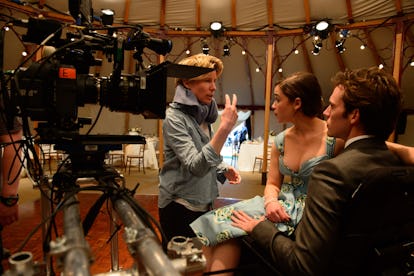In a tented film set with white walls and a brown wooden floor, a blonde female director in a blue button-down shirt, with earphones slung around her neck, engages two actors. The director holds two fingers near her face, mid-gesture, as she speaks to a man in a brown suit and a woman in a low-cut blue dress seated on his lap. The man has light brown hair, while the woman has short brown hair, with her right hand resting on her dress. A large black camera, laden with wires and mounted on two metal poles, stands to the left of the director. Overhead, lights are strategically positioned, illuminating the scene. In the background, tables and chairs suggest a possible wedding scene, completing the detailed ambiance of this film set.